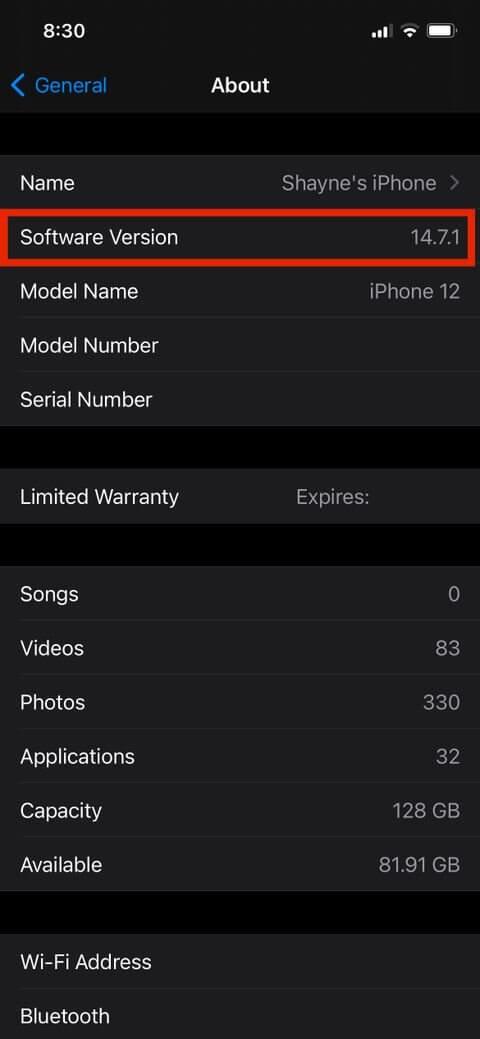The image presented is a screenshot taken from an iPhone, specifically displaying the "About" section within the device's settings. The distinctive layout and font confirm it's an iPhone, showing details typical for this setup screen.

The time displayed at the top of the screenshot is 8:30, and the battery icon indicates a charge level close to 100%, probably around 90-95%. The network symbols show a strong Wi-Fi connection and cellular signal. The device is currently set to dark mode.

Information listed in the "About" section includes:
- **Device Name:** Shane's iPhone
- **Software Version:** iOS 14.7.1
- **Model Name:** iPhone 12
- **Storage Capacity:** 128 GB 
- **Available Storage:** 81.91 GB
- **Media Stored:**
  - **Songs:** 0
  - **Videos:** 83
  - **Photos:** 330
  - **Applications:** 32

Details like the serial number, limited warranty expiration, Wi-Fi address, and Bluetooth address are not displayed in the screenshot.